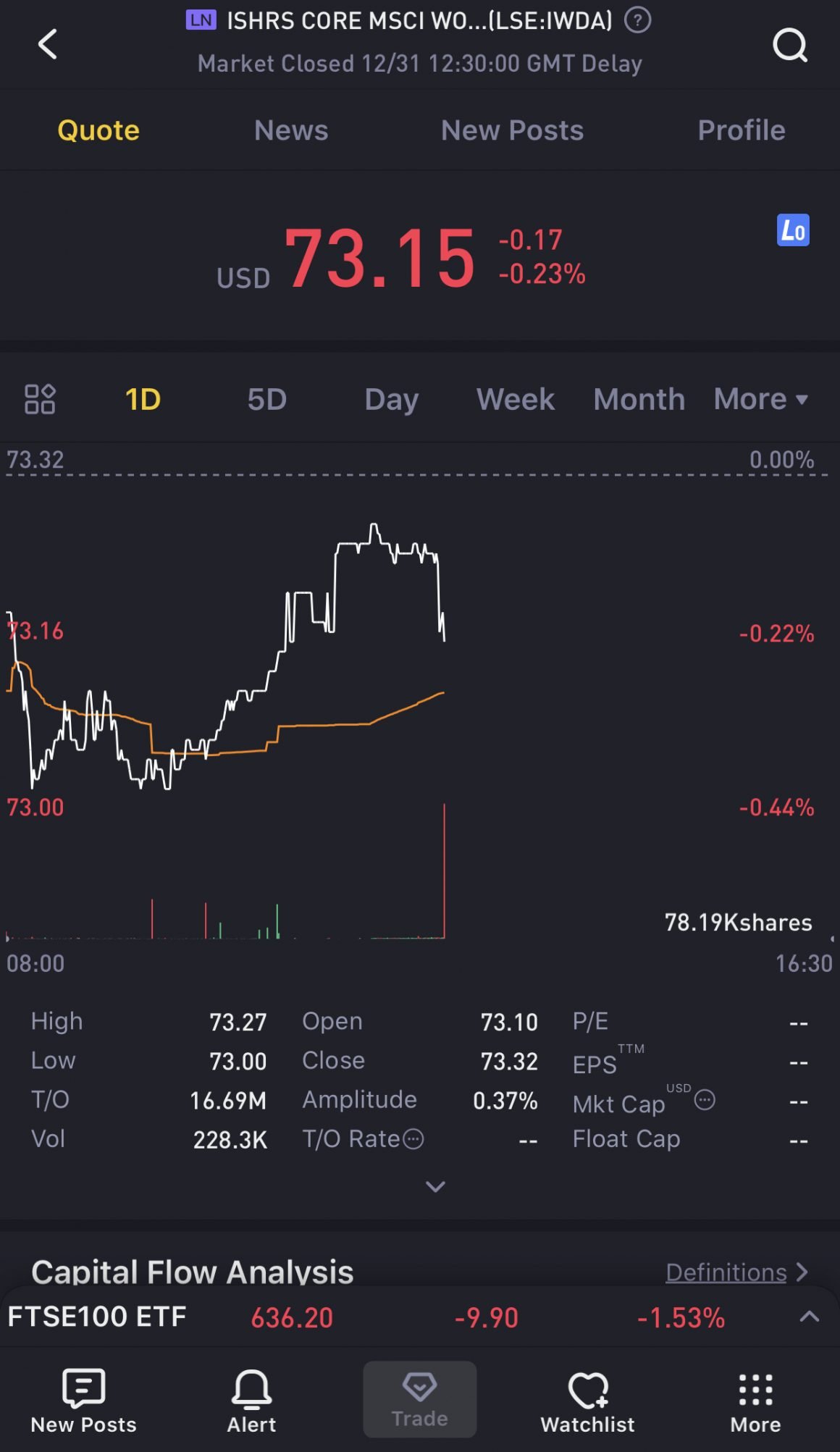This screenshot captures an interface of a stock tracking app. At the top of the screen, the current value of a stock is prominently displayed at 73.15 USD. This stock is identified as "ISHRS Core MSCI" in the header section. Beneath this, a status message denotes "Market Closed" with a timestamp of "December 31st, 12:30 GMT" and indicates data delay.

The app features several navigational tabs positioned just below the stock name, arranged from left to right: "Quote," "News," "New Posts," and "Profile." The "Quote" tab is currently selected, highlighted in yellow. Below the stock value, additional tabs for different time frames are presented: "1D," "5D," "Day," "Week," "Month," and "More." These likely represent different periods for viewing stock performance, with "1D" for one day, "5D" for five days, "Day" for the current day, "Week" for a week, and so forth.

Prominently displayed beneath these tabs is a dynamic graph charting the stock's performance. The graph shows significant fluctuations: an initial decline followed by a rise, a sharp drop, a pronounced recovery, and another dip. The latest data points indicate that the stock is currently down by 0.22% from its value at the start of the day, sitting below the 0% mark.